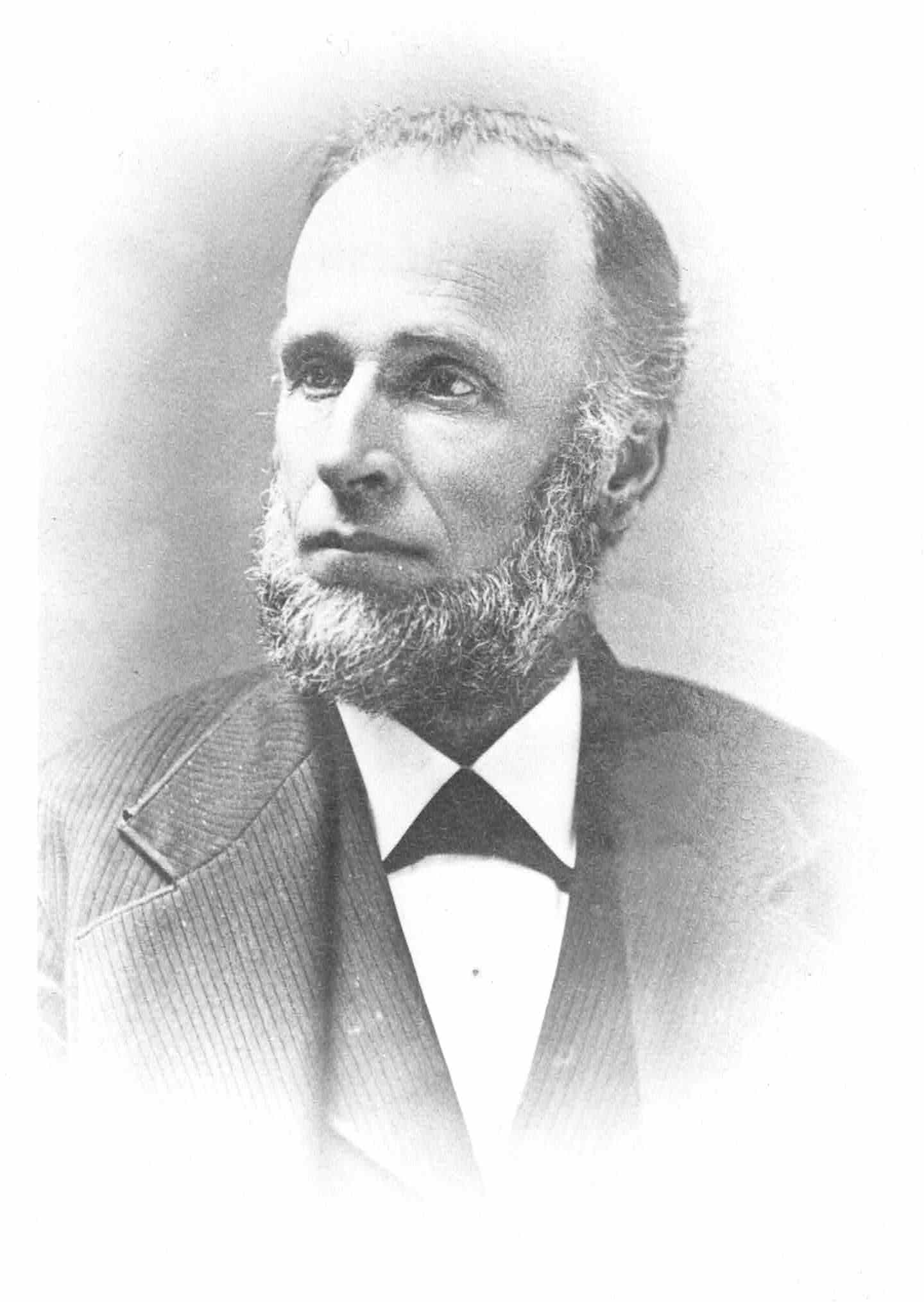This black and white photograph portrays a distinguished man, possibly from the late 1800s or early 1900s, attired in a neat and tidy suit. He is wearing a dark blazer, which appears to have pinstripes, along with a matching vest. Underneath, he sports a buttoned-up white collared shirt accompanied by a black kerchief or tie at the neck. His head and shoulders are central to the image, with his head turned slightly to the left, away from the camera, allowing a side profile of his face. The gentleman has a beard that connects seamlessly with his sideburns and short, neatly-parted, brushed-back hair that might once have been brown but now shows signs of graying into a salt and pepper look. He bears a few noticeable wrinkles on his forehead, suggesting he is in his 50s. The overall impression is of a person of importance, potentially a professor or a figure in politics, given his composed and dignified appearance.